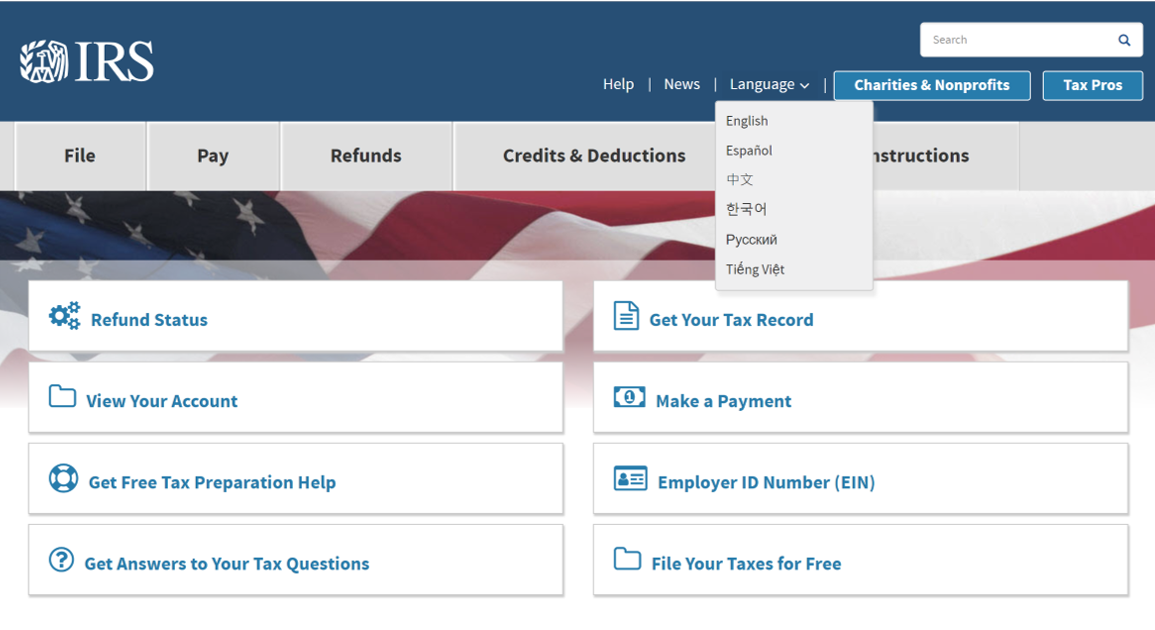This image is a detailed screenshot of the IRS website homepage. At the top of the page, a prominent blue banner features the IRS logo, flanked by navigational links labeled “Help,” “News,” “Language,” “Charities & Nonprofits,” and “Tax Pros.” Below this, another horizontal menu provides options for “File,” “Pay,” “Refunds,” “Credits & Deductions,” and “Instructions.”

The background features a waving American flag, giving a sense of national identity and pride. Centrally positioned are eight clickable buttons arranged in two columns and four rows. The buttons are white with blue text and icons, offering the following services:

**Left Column:**
1. **Refund Status** – Check the status of your tax refund.
2. **View Your Account** – Access and review your tax account.
3. **Get Free Tax Preparation Help** – Obtain assistance with tax preparation at no cost.
4. **Get Answers to Your Tax Questions** – Find answers to common tax-related queries.

**Right Column:**
1. **Get Your Tax Record** – Retrieve your tax records.
2. **Make a Payment** – Make tax payments online.
3. **Employer ID Number** – Apply for or retrieve your Employer Identification Number.
4. **File Your Taxes for Free** – Submit your tax returns without any charges.

Additionally, the language drop-down menu is expanded, showing six language options: English, Español, and several others, among which Vietnamese and Russian are tentatively identified.

Overall, the screenshot provides a comprehensive view of the IRS website’s home page, highlighting its user-friendly design aimed to facilitate various tax-related tasks.